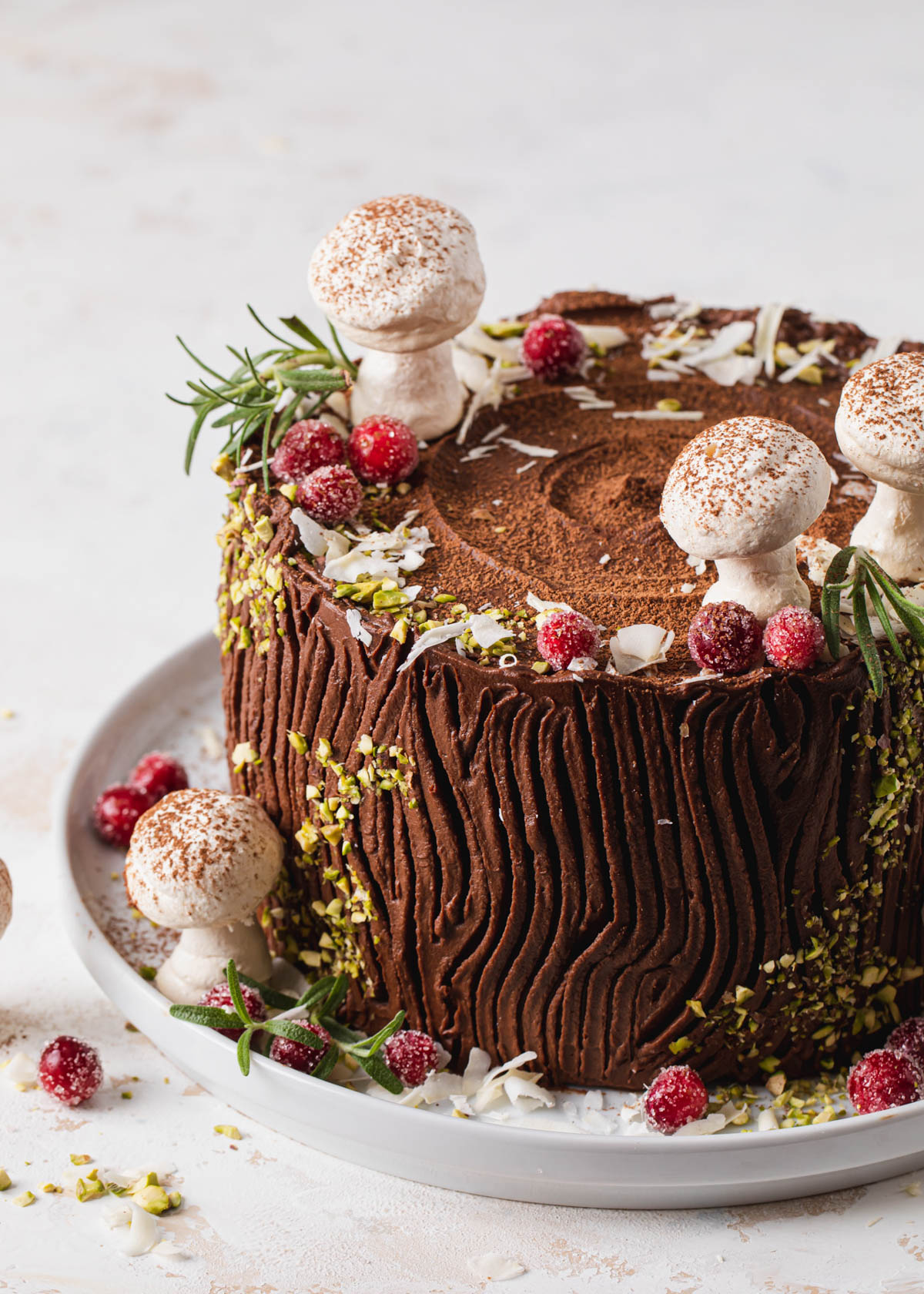This photograph showcases an intricately designed cake inspired by nature. The cake, artfully shaped and textured to resemble a tree log, features a rich brown chocolate icing with detailed patterns mimicking tree bark. Topping the cake are delicate, edible structures crafted to resemble white mushrooms, adorned with cocoa powder to imitate brown speckles. Vibrant red, sugar-coated berries are scattered across the cake, adding a pop of color and festive touch, while fine shreds of coconut enhance the woodland theme. Green elements, likely chopped pistachios, decorate the sides of the cake to resemble algae or moss. This edible masterpiece is presented on a shiny, round white plate, made of glass or ceramic, set against a pristine white background.